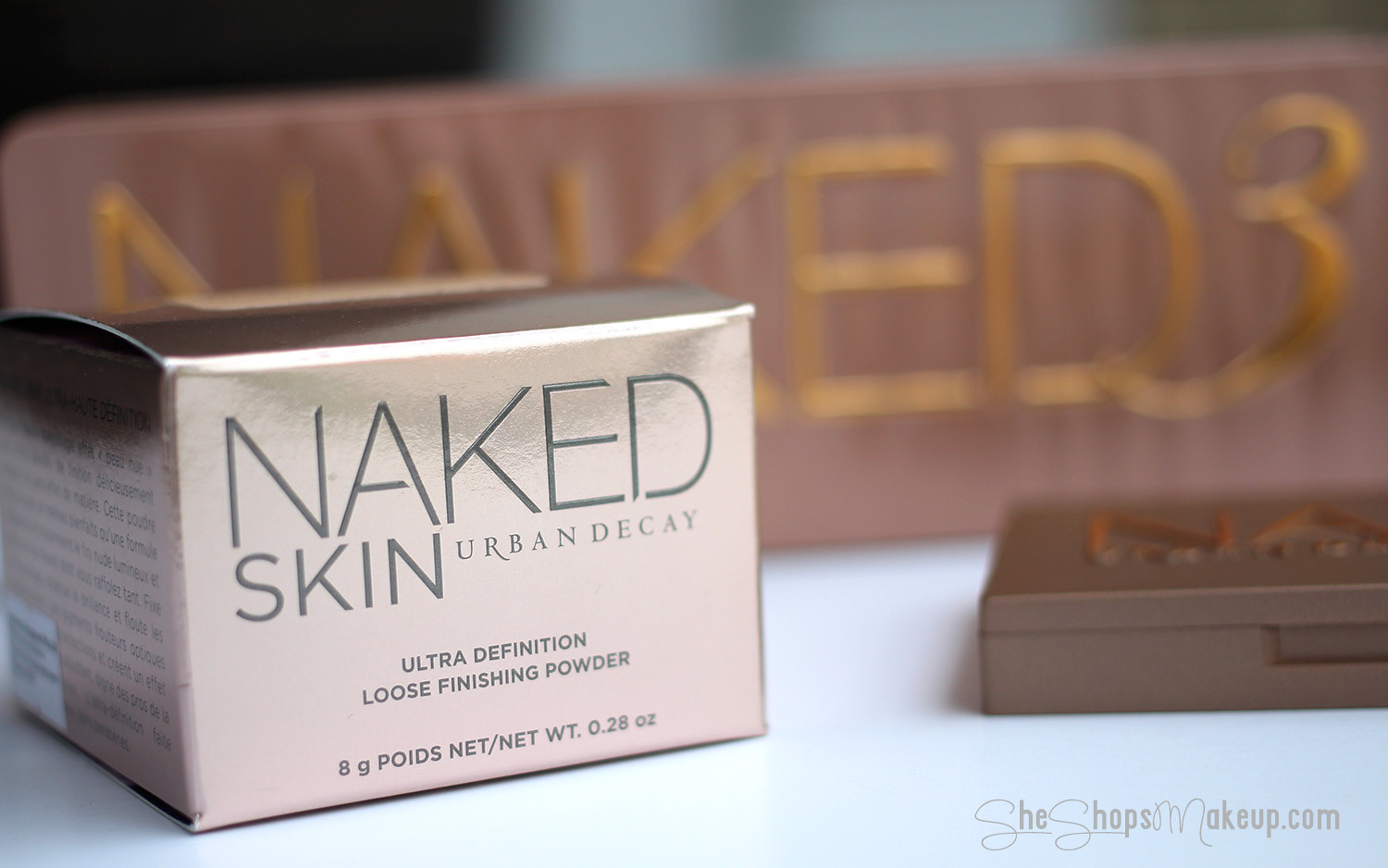The image showcases a box package of a skin care product set against a light blue surface. The skin care product's box is on the left side of the image, featuring a light pink or possibly gold metallic hue. The most prominent word on the front of the box is "Lacked," with "Skin" following closely in size, both in large black letters, and the smallest print reads "Urban Decay." Below, the description states, "Ultra-Definition Loose Finishing Powder," with the net weight listed at the bottom as "80g POIDS Net / 0.28 oz." The box is slightly turned to the right, revealing additional black text on its side.

Adjacent to the box, on the right, there is a thin, flat brown plastic container. The container shows engraved letters "A" and "N" in gold on its top surface. Behind these items, a plaque with gold lettering stands out, displaying "Naked 3," hinting at a display for the Urban Decay Naked Skin product line. In the bottom right corner of the image, there's a faint website link: "SheShopsMakeup.com," potentially indicating the retailer for this product.